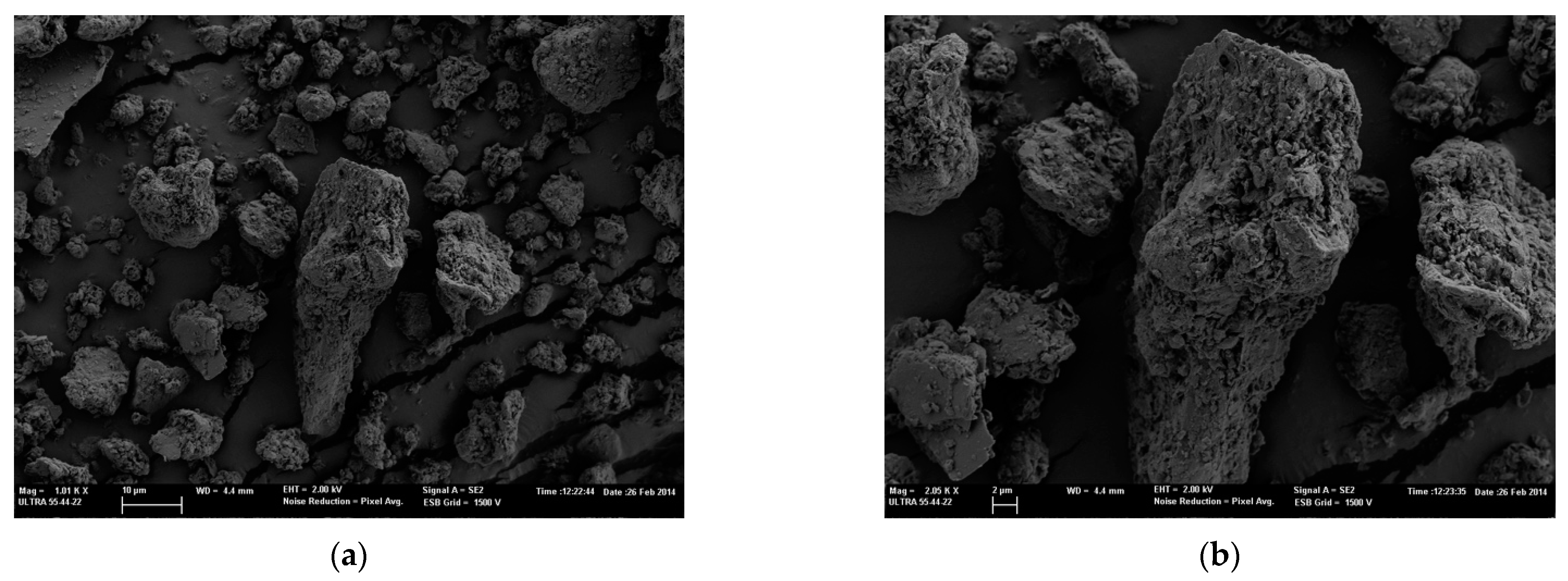The image consists of two black-and-white microscopic photos. The one on the left shows a highly magnified smooth surface with numerous, irregularly shaped rocky formations of various sizes scattered across it, all intersected by numerous cracks. This image is accompanied by a timestamp reading "12:22:44" from February 26, 2014, along with text detailing scientific data such as noise reduction, pixel average, signal A, and ESB grid. The image on the right is a further magnified view of the same area, focusing closely on the central largest rocky formation flanked by two large stones. This zoomed-in photo includes a timestamp of "12:23:35," indicating it was taken approximately a minute after the first. The detailed, crack-covered texture and the arrangement of the formations suggest that this could be a close-up study of a geological surface.